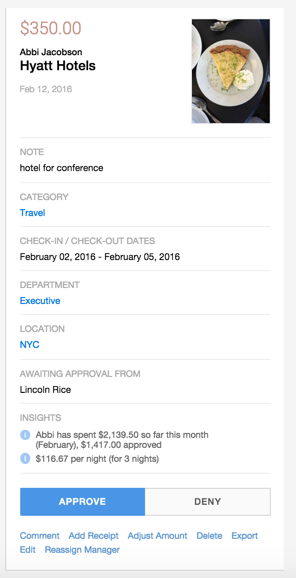This image presents a detailed view of a page filled with various pieces of information. In the top right corner, there is a slice of pizza served on a plate, adding a casual touch to the otherwise formal content. On the top left, the text reads "$350, a big check-up scene, Hyatt Hotels, February 12, 2016," suggesting an expense or reimbursement related to a hotel stay. Below this text, a section delineates specific details: "Notes, hotel for conference, category travel, check-in and check-out dates from February 02, 2016 to February 05, 2016."

Further down the page, we see a segment that appears to list tasks. The first task is dated Saturday, the 28th, and includes an option to add a task labeled "observations." Another entry, scheduled for Monday, November 14th, signifies an event or deadline, indicated by the phrase "it's here." Additional details outline instructional activities such as "Instructional round sign-ups," "give us reading scope and sequence," and "follow up grade 4 to 5." This comprehensive and structured page likely serves as a planner or an organized collection of professional activities and notes.